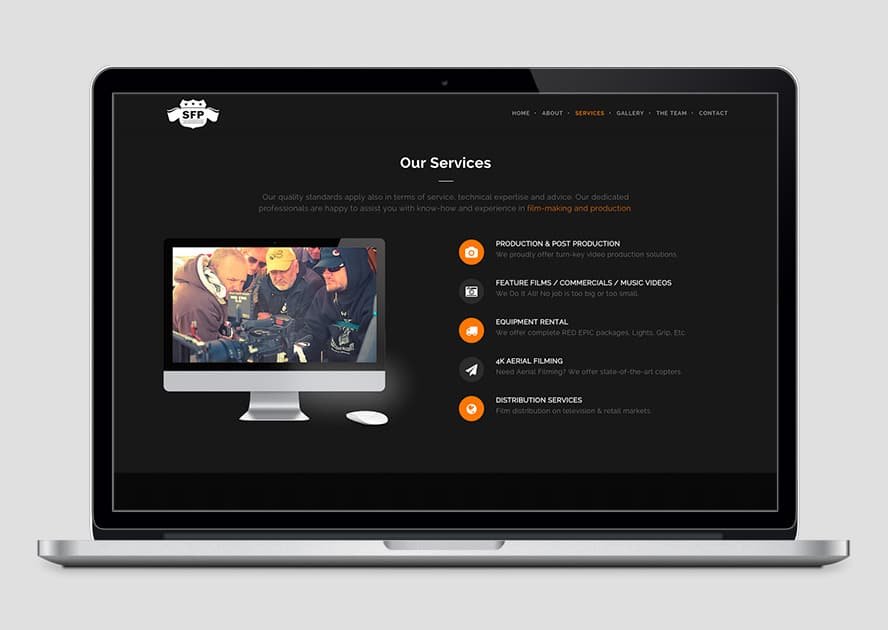The image depicts a laptop with a sleek, bright silver metallic frame. The screen, outlined by a black border, displays a website against a light smoke gray background. In the top-left corner of the screen, there's a white shield-like icon featuring the letters "SFP." 

Below this icon, a gray and black computer monitor image is displayed, accompanied by a small mouse which appears white or silver. The section titled "Our Services" is prominently shown with relevant information beneath it.

On the right side of the screen, there are five icons: three in orange and two in a grayish-black color, representing functions such as a camera, sending a message, and other utilities. The top-right corner of the screen contains navigation tabs for exploring different sections of the website.